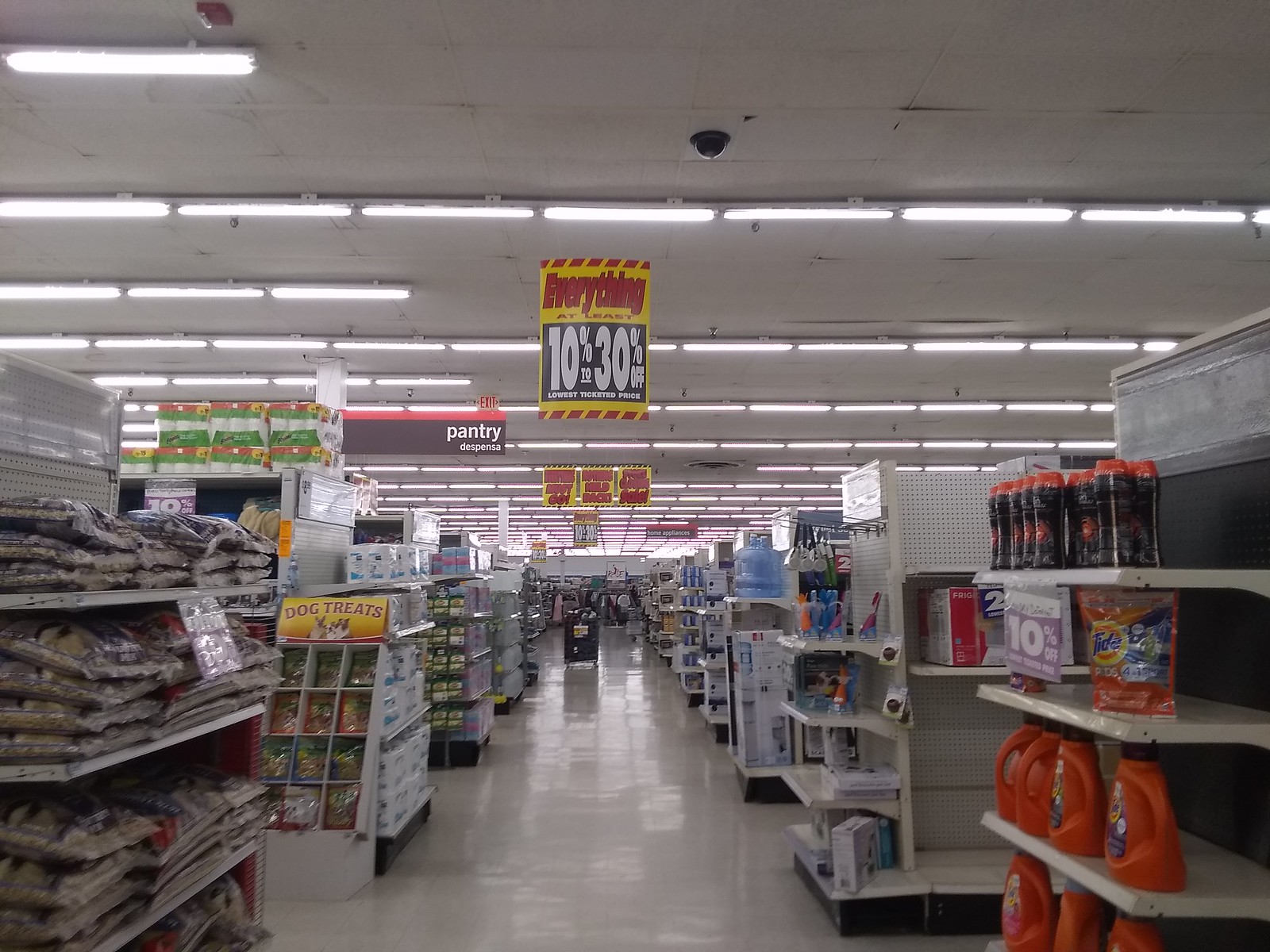This photograph captures a store interior with an aisle running straight down the middle, providing a clear view of the entire store-length. The ceiling of the store is white and features a black security camera prominently positioned. The ceiling also hosts a series of white lights, some of which span the entire width while others are segmented into groups of three.

A notable element in the photograph is a large banner located centrally, featuring a combination of yellow, red, white, and black colors. The banner displays "10 something 30" along with additional red lettering. 

The aisles are lined with white shelves, and in the bottom right corner, orange laundry detergent bottles are visible. Across from them, on the left side, there appear to be candy items. The store's flooring is also white, adding to the brightness of the scene.

A sign indicating "pantry" is visible, characterized by white lettering on a black background with a red stripe at the top. This image appears to have been taken in a dollar store or a discount store, although no specific store name is visible. The overall tone of the image is slightly dark.